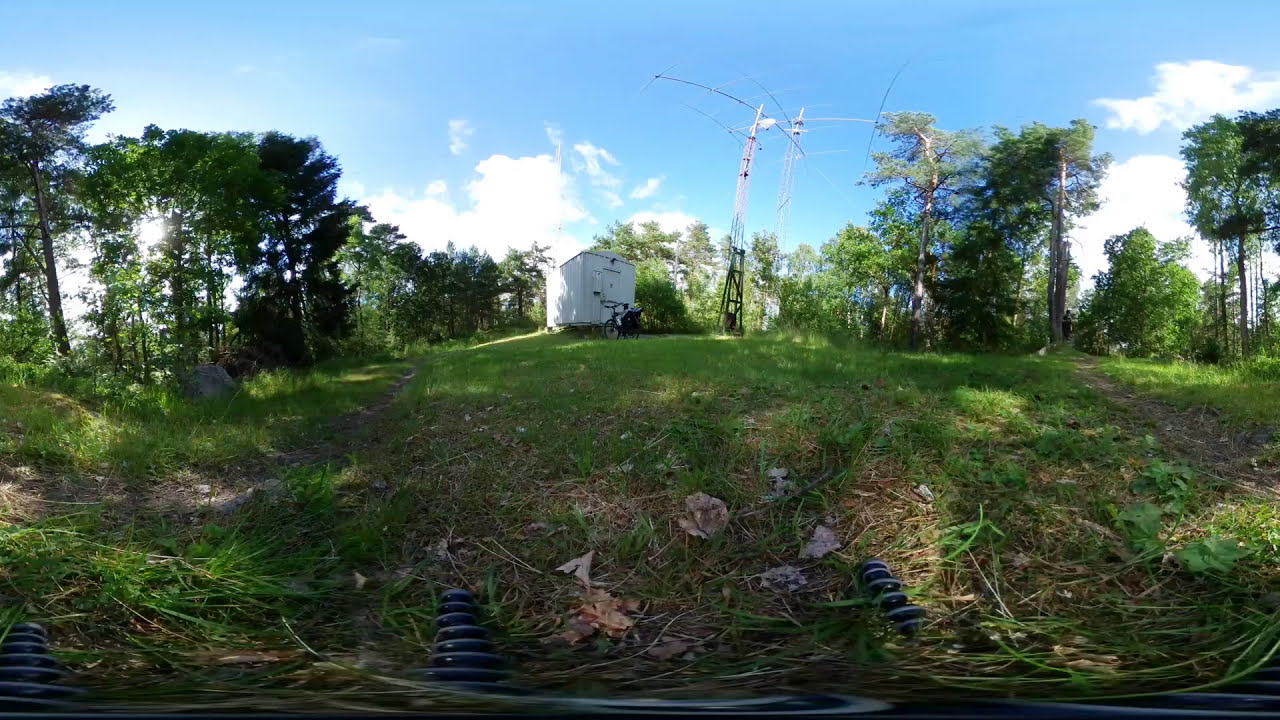In the photograph captured on a sunny, bright day with a vibrant blue sky and scattered white clouds, we observe a small grassy hill topped with a variety of technological structures. At the base of the hill, scattered across the green grass and amidst leaves, are round, tubular knobs that appear to be out of place, possibly remnants of some electrical equipment. These black and gray coils form a horizontal pattern that spans from one side of the image to the other, giving the impression that multiple images were stitched together, resulting in a slightly warped, fisheye effect.

Ascending the grassy hill, we encounter several tall, white towers that resemble radio or communication towers, complete with arms extending outwards adorned with dipoles. These towers are flanked on the left by a white shed or cabin, which has a bicycle propped up against it. To the right, a person can be faintly seen standing near a tall tree, adding a human element to the otherwise technological landscape. The backdrop of the scene features lush green trees with sunlight filtering through the leaves, creating a serene and lively atmosphere.